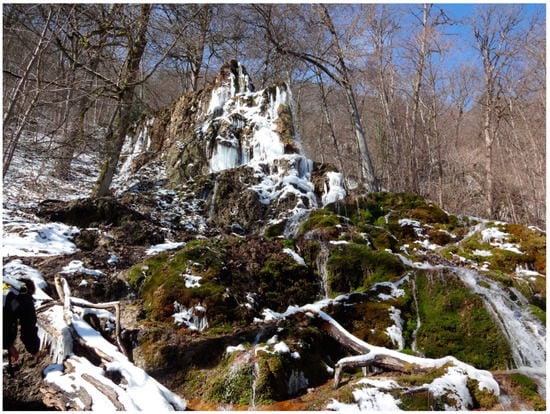The image depicts a picturesque winter scene featuring a small, frozen waterfall nestled in a mountainous area. The photo is taken from a hillside, looking upwards, capturing a clear blue sky framed by the bare, leafless branches of numerous thin trees. The ground is lightly snow-covered, particularly on the left side, where patches of dirt and grass also emerge. At the centerpiece, there's a mound or ledge of rocks adorned with green moss and brown hues. Water appears to be cascading down from a higher plateau to a lower one, with some portions seemingly frozen in mid-flow, contributing to the wintery atmosphere. Scattered tree roots and branches, some covered in snow, add texture to the foreground. Overall, the landscape showcases a blend of whites from the snow, browns from the rocks and trees, greens from the moss and ground foliage, and blues from the sky, offering a serene and natural snapshot potentially captured by someone exploring the wintery outdoors.